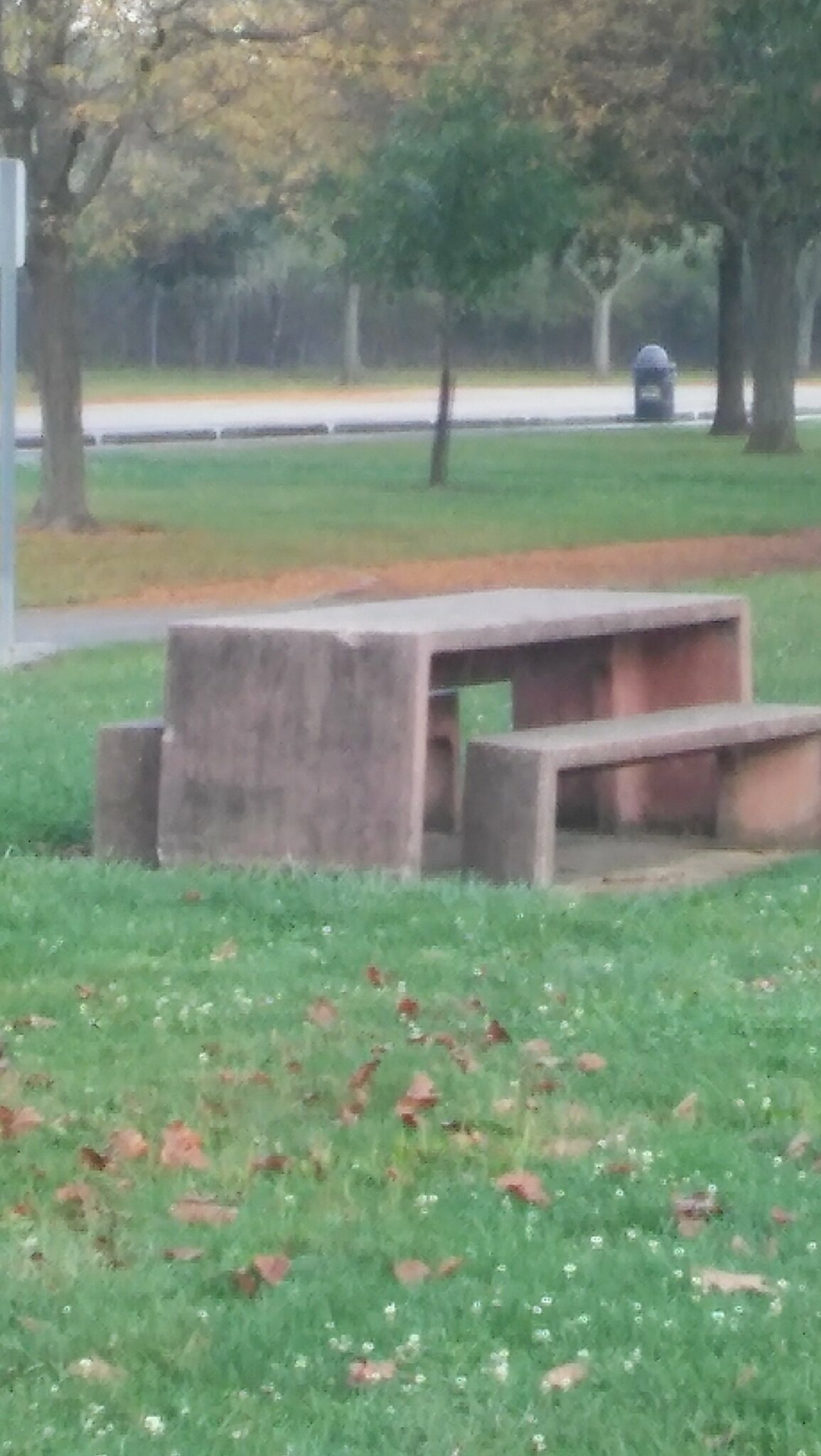The photograph captures a serene park setting featuring a cement picnic table with matching benches positioned on a small concrete pad amidst a grassy area. Sparse autumn leaves are scattered across the grass in the foreground. Behind the table, there is a dirt patch flanked by four trees, leading to a partly visible parking lot marked by empty spaces and a trash can in the upper right corner. Beyond the parking lot, a gray chain link fence is discernible, with a thick tree canopy occupying the top section of the image. The trees display early fall colors, adding a touch of seasonal charm to the scene. Small white flowers, possibly daisies, and a few brown leaves are dotted around the grass, completing the picturesque view.